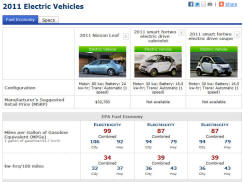This is an image from a website dedicated to electric vehicles, although it is heavily compressed and blurry. The background is solid white. In the top left corner, there's bolded blue text that reads "2011 Electric Vehicles." On the right side, a blue wire extends from right to left, followed by an orange square and a vertical black line. There are three other indiscernible icons beside these, followed by a recognizable Facebook icon.

Below the "2011" text, a blue tab with unreadable white text is visible, next to a white tab with black, also unreadable, text. A thin dark blue border runs horizontally across the width of the image beneath these tabs. Beneath this border is an empty white square with illegible black text below it, followed by a line and two more lines of unreadable black text.

To the left of this section are three car images: a blue car facing left, and two smart cars—the middle one facing left and the right one facing right. Above the cars, there is additional blurred black text, and green tabs with white, unreadable lettering are located directly above one of the cars. Below the cars are several lines of black text, all unreadable.

The lower portion of the image features a gray border with black text in the center, also unreadable. On the left side, there are two lines of illegible black text, with another rectangular section below containing more unreadable lettering. To the right of each of these sections are three boxes containing letters and numbers, which remain indiscernible due to the blurriness.